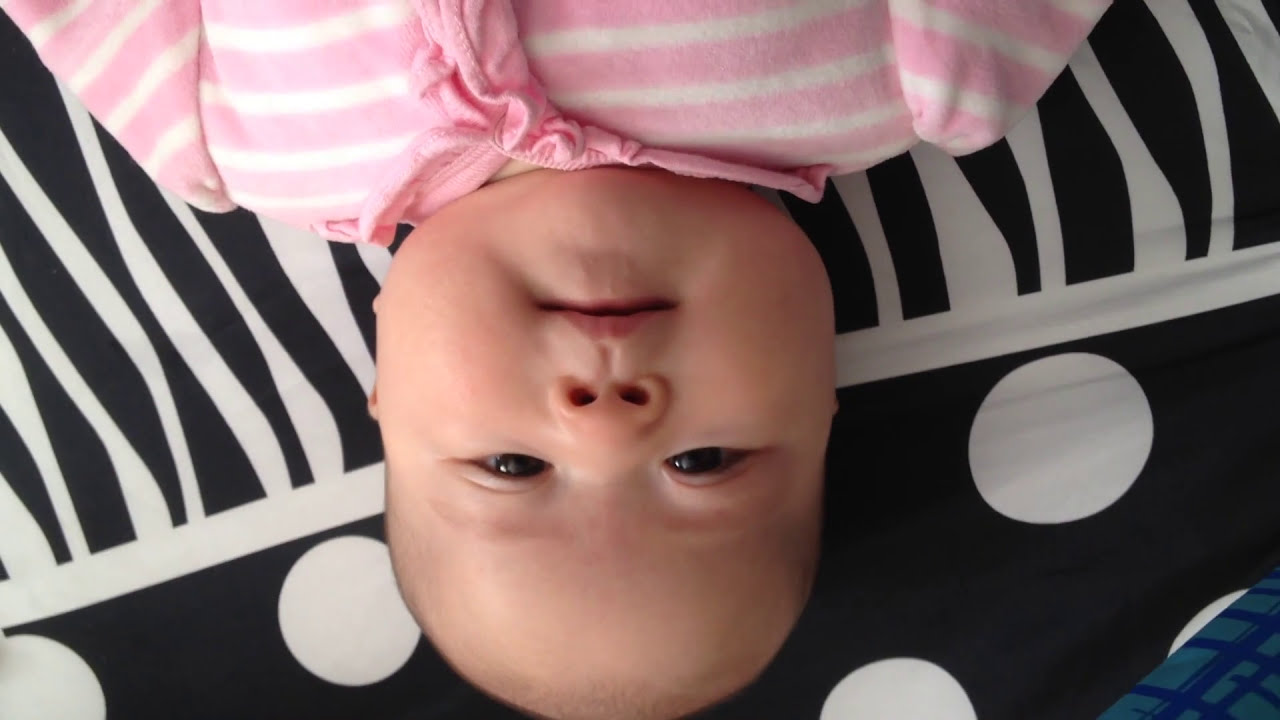In this image, a baby girl with medium olive skin tone is lying upside down on a bed, gazing up into the camera with her mouth shut and eyes open. She has chubby cheeks and little to no hair on her head. Dressed in a soft pink and white striped onesie, she is positioned at the center of the photo, highlighted against a backdrop of distinct patterned fabrics. The bedding features black and white polka dots in the middle, a zebra-like design at the bottom, and an edge of dark blue and light blue patterns on the far right. The indoor setting, possibly a crib, emphasizes the unique perspective and central focus on the upside-down baby girl.